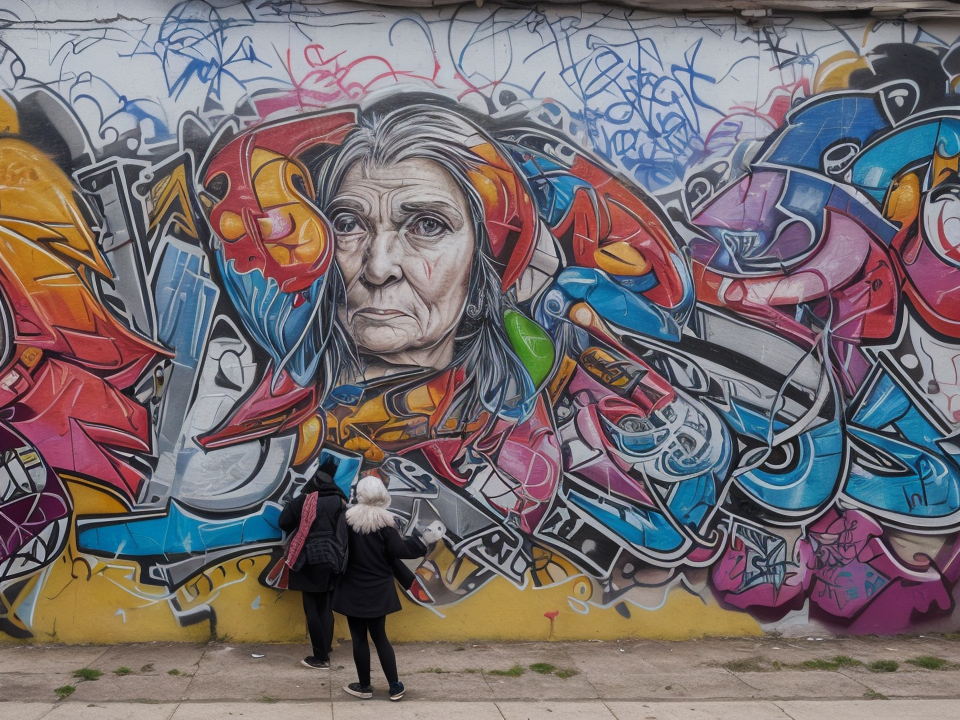The photograph captures a vivid street scene where two people, both dressed in black jackets, black pants, and black sneakers with white soles, stand on a sidewalk, engrossed in viewing a large, vibrant mural on the side of a building. One person, who has white hair or is wearing a light-colored head covering, is on the right, while the person on the left carries a red or pink bag or scarf over their left shoulder. The mural's main focus is the face of an older woman with a wrinkled visage and white hair that seems to blend into the surrounding abstract and graffiti-style artwork. Her face, with tiny lips and intriguing eyes—one appearing normal and the other split like it has two pupils—is set against a colorful backdrop of reds, blues, pinks, purples, and yellows. These colors intermingle with various abstract shapes and graffiti tags, creating a dynamic and layered visual effect on the white base wall. The bottom section of the mural features a yellow hue, with some green algae patches visible on the sidewalk below. To the right of the woman's face, there is a depiction that resembles the eye of a creature, while to the left, a head of a snake with an open mouth can be seen. Bold black outlines punctuate the overall vibrant composition of the artwork. The photograph captures the essence of urban artistry and the intrigued observers appreciating its complexity.